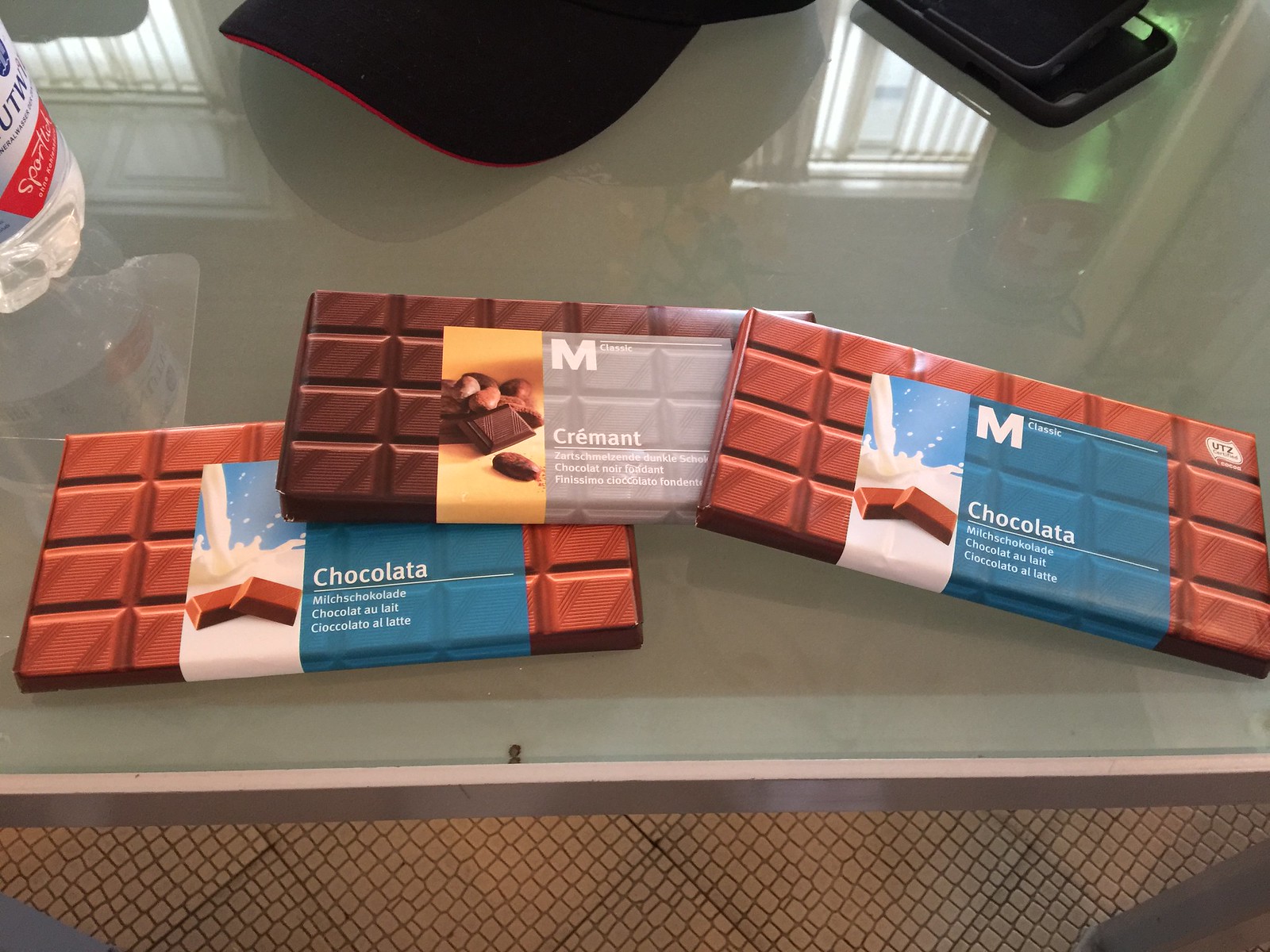The image features three Swiss chocolate bars prominently displayed on a highly glossy, possibly glass, countertop with a pearlized, whitish finish. These chocolates, labeled "M Classic," are flavors of Chocolata Milchschokolade (milk chocolate), a darker Cremant, and another Chocolata. The milk chocolate bars, wrapped in light brown packaging, are identical, while the Cremant bar is in a darker brown wrapper and positioned diagonally. The countertop is set against a textured floor in shades of brown and black, suggesting a retail environment. To the left of the chocolates, there’s a bottle of water and a baseball hat. A green-lit phone is also visible, adding a touch of technology to the setting. The clear, reflective surface of the countertop even shows the reflection of the water bottle, adding depth to the scene.